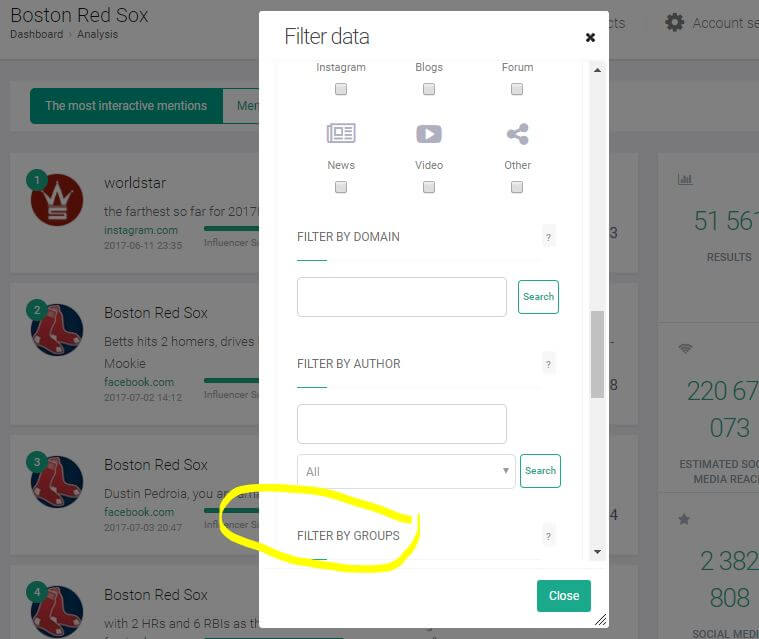This image showcases the Boston Red Sox website, prominently featuring a central pop-up tab. The background appears grayish, typical when a pop-up tab is active. 

In the upper left corner, the text "Boston Red Sox" is displayed in black. Just below, the options "Dashboard" and "Analysis" are listed, also in black. 

On the right side, partially obscured by the pop-up tab, there is visible text "CTS" along with a settings icon, accompanied by a partially visible "SE" counter extending off the edge. Below this, a green tab bears the white text "Most Interactive Mentions," and beneath it, a white tab displays green lettering reading "ME."

The page contains four small rectangular sections, each featuring a circular profile picture. The first section is titled "World Star," while the subsequent three sections are all related to the Boston Red Sox. Each rectangle includes a green circle in the top-left corner displaying sequential white numbers (1, 2, 3, and 4).

The central pop-up is approximately four inches wide, with a white background. At the top, "Filter Data" is written in black, accompanied by a black 'X' on the right side for closing the pop-up. Below "Filter Data," various filter categories are listed: "Instagram" with a gray square underneath, "Blogs" with a corresponding box, "Forum," "News" with a newspaper icon, "Video" with a YouTube icon, and "Other" with a share icon. 

Additional filtering options include a search bar labeled "Filtered by Name," another one "Filtered by Author," and a general search bar marked "All" with a "Search" button next to it. The section "Filter By Groups" is highlighted in yellow.

In the bottom right corner, there's a blue button with white text that says "Close."

The right side of the pop-up shows a list of numbers: 51, 56, 202, 067, 073, with some numbers continuing off the page. At the bottom, numbers such as 2382 and 808 are partially visible.

This detailed description encapsulates the intricate elements of the Boston Red Sox website as seen in the image.